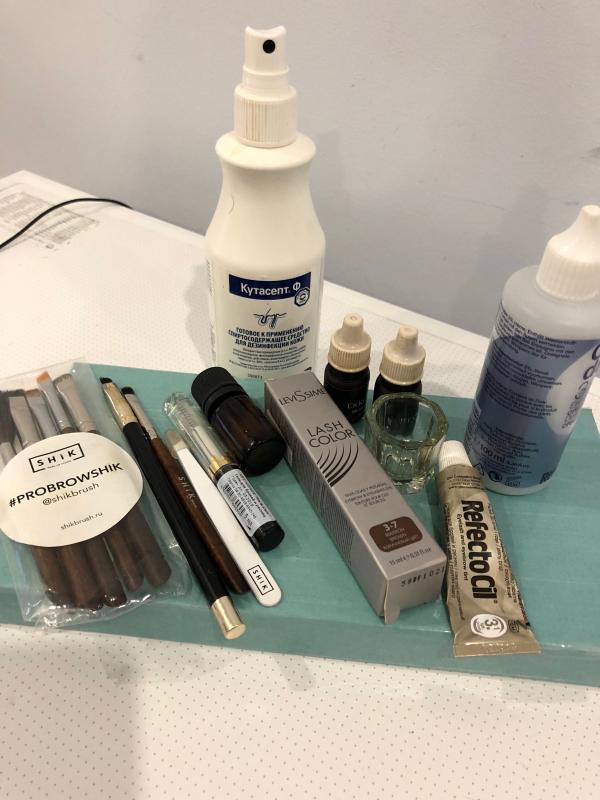The photograph features an assortment of makeup items and beauty products carefully arranged on a turquoise slab, which is set on a white plastic table. Dominating the composition are two significant bottles: one is predominantly white and equipped with a push-down spray nozzle, though its label is unreadable. Beside it, there is a clear bottle wrapped in blue packaging, capped with a white, pointed screw top, the contents of which are also indiscernible.

In addition, a golden tube resembling a toothpaste container is prominently displayed. The tube, labeled "RefectoCil," hints at its beauty-related nature, though the exact product is unspecified. Accompanying these items, a long, rectangular silver box with the partial inscription "Levy something lash color" suggests it might be mascara. 

Lastly, an assortment of makeup brushes is neatly packed inside a transparent plastic bag, marked with a white circular label that bears the brand name Schick and the hashtag #ProBrow. These meticulously placed items offer a glimpse into a variety of beauty and makeup essentials.